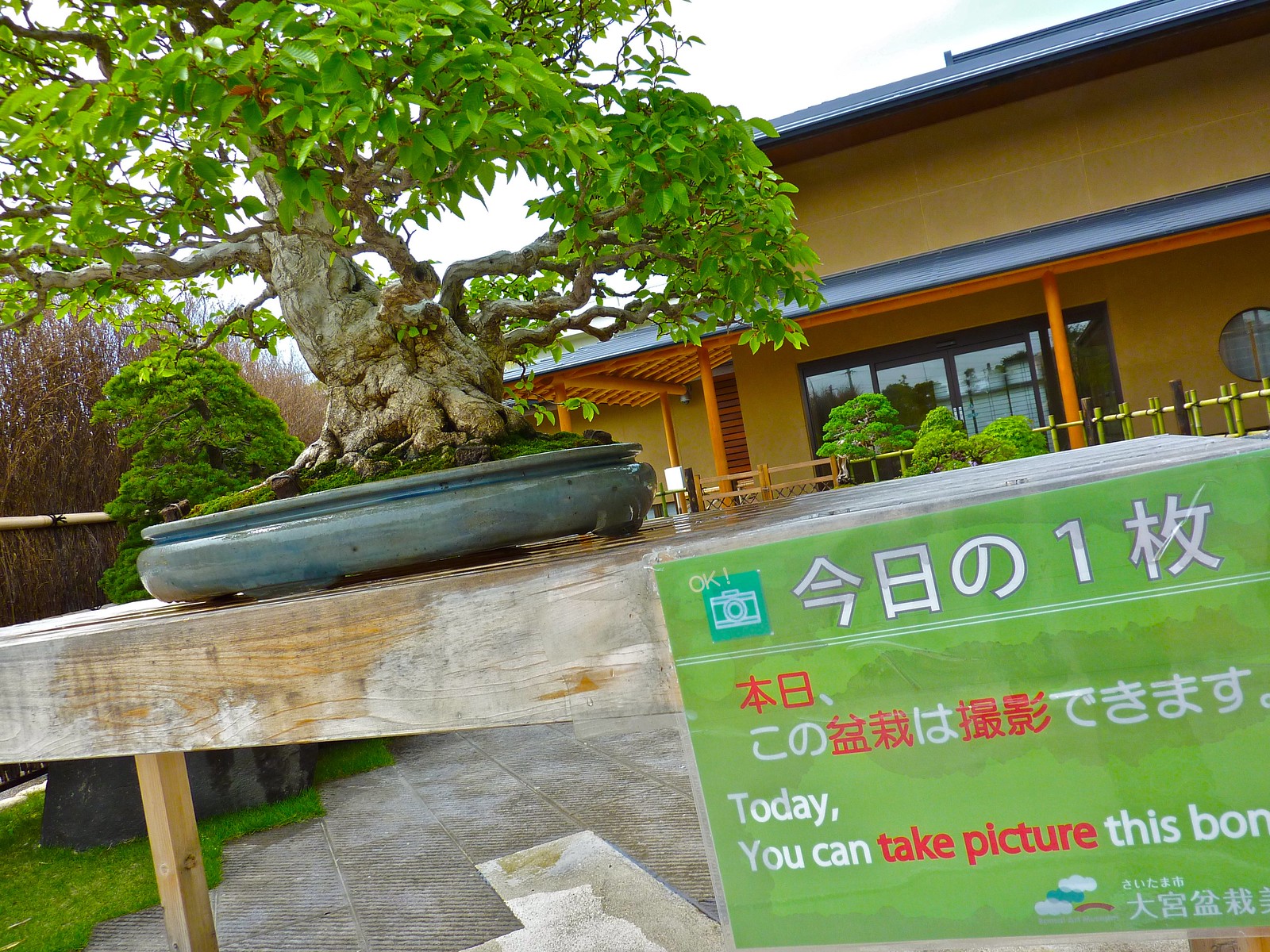The photo captures an outdoor scene with a close-up of a worn, aged wooden table. On this table sits a large, very green bonsai tree in a black pot. There is a green laminated banner stapled to the front of the table, featuring foreign writing—possibly in Japanese or Korean. Beneath the foreign text, a partly cut-off English translation reads, "Today, you can take picture this bonsai." Flanking the right side of the table, a small dish can be observed. The setting includes a concrete patio leading to a garden space with some greenery and trees, including a spruce tree to the left. In the distant background, a yellow and beige building with orange pillars holding up an overhang and a large picture window can be seen, contributing to the serene backdrop of the scene.